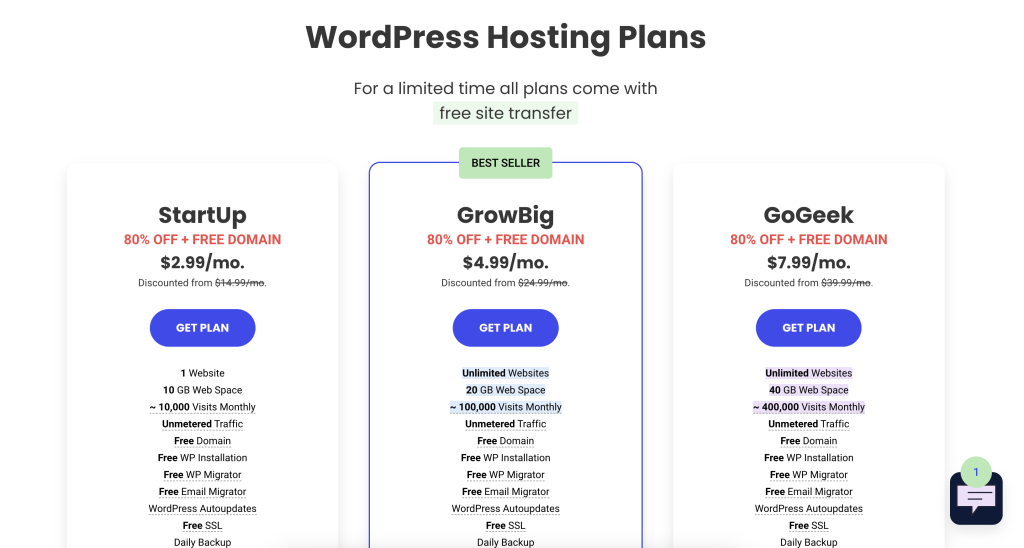The image showcases various pricing plans for WordPress hosting services. It is wider than it is tall, with a predominantly white background. 

At the top, in black text, it states "WordPress Hosting Plans," indicating the offer pertains to hosting solutions for websites built on WordPress.org. Below this heading, in green text, it highlights a limited-time offer: "For a limited time, all plans come with free site transfer."

The pricing plans are divided into three tiers: 

1. **Startup**:
   - Priced at $2.99 per month, discounted from $14.99.
   - Accompanied by a blue "Get Plan" button.
   - Details of what the plan includes are also provided, albeit not specified in our description.

2. **Grow Big** (marked as the bestseller):
   - Offered at $4.99 per month, reflecting an 80% discount.

3. **Go Geek**:
   - Available for $7.99 per month.

In the bottom-right corner of the image, there's a black square icon with rounded corners. Inside this icon, there is a lavender text message symbol featuring the number 1 in a circle.

This image appears to be promotional material from a web hosting company offering discounted rates for hosting WordPress websites, including an additional perk of free site transfers for a limited time.